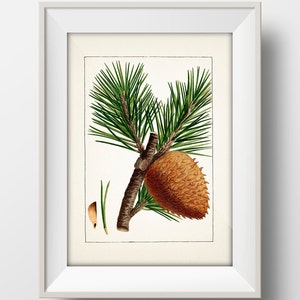The image is a realistic, square photograph of a framed picture hanging on a beige wall. The frame is white, wooden, and beveled, approximately one and a half to two inches wide. Inside, an off-white matting surrounds the picture. The central piece appears to be either a hand-drawn or computer-generated rendition of a pine tree branch. The main subject includes a short, wide, brown pine cone hanging from a green, woody branch, which extends into two smaller branches adorned with clusters of green pine needles. To the left of the main branch, a detailed sketch shows a close-up of one or two individual pine needles and a single segment of the pine cone, set against a white background to highlight these elements. The composition provides an intricate view of the pine tree, with careful attention to the textures and details of the needles and cone.